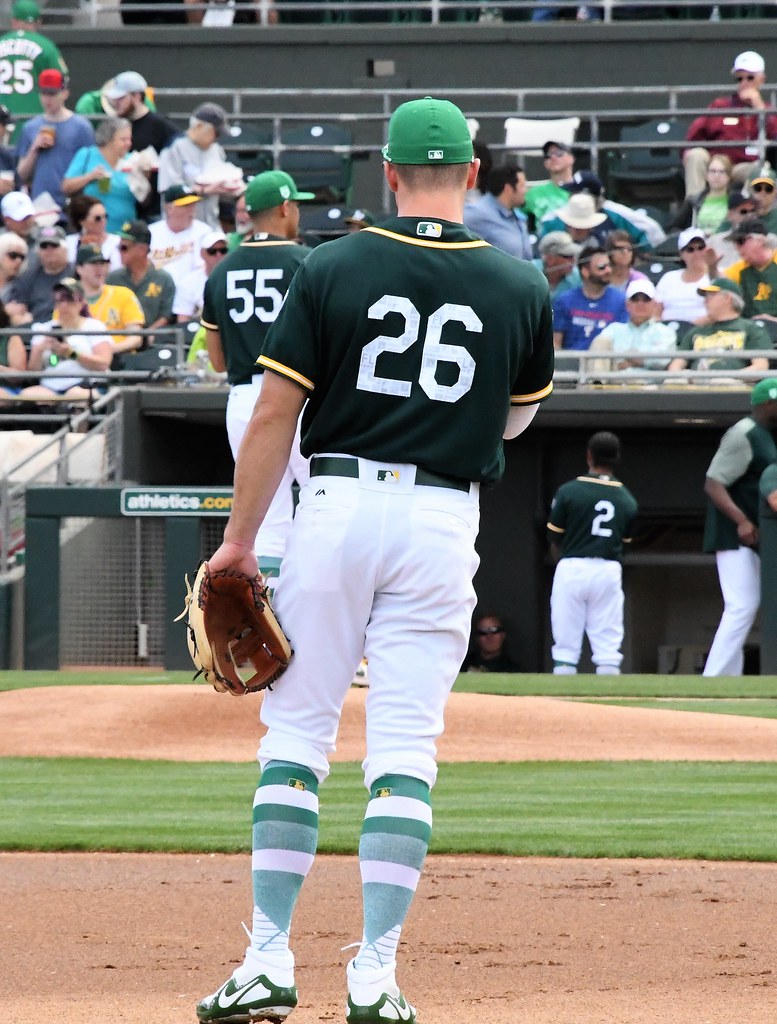The image captures a vibrant scene at a baseball game, featuring both players and fans. The central focus is on a player with the number 26, dressed in a dark green jersey with yellow accents, white pants, green belts, green and white striped socks, and white cleats bearing a green Nike check. He is holding a baseball glove and facing the grandstands, which are filled with spectators dressed in a variety of colors such as red, blue, maroon, white, green, and yellow. Prominently visible alongside him are players number 55 and number 2, wearing similar green uniforms. The backdrop reveals three levels of grandstands, though the third level is only partially visible. Fans in the stands are seen walking around, some holding food, contributing to the lively atmosphere. A sign in the bullpen reads "athletics.com," indicating the team's association.